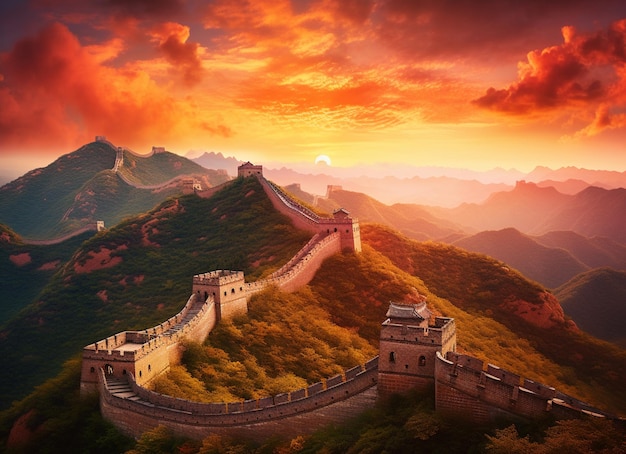The image is an artistic representation, likely a painting, of what appears to be the Great Wall of China extending through a vast, mountainous landscape. The scene is suffused with the warm hues of a sunrise or sunset, featuring an orange, yellow, and deep red sky with a few clouds adding texture. The mountains and hills are richly green, and the wall, which appears tan or beige due to the sunlight, crisscrosses over them, disappearing into the horizon. The wall includes numerous towers, each detailed with crenelated tops and windows, contributing to its majestic architecture. The light from the sky casts intricate shadows and illuminates the wall and mountains in a striking manner, heightening the fantasy-like quality of the image. No people are visible, emphasizing the grand scale and serene atmosphere of the landscape.